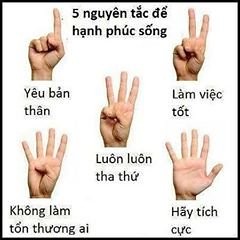The image depicts a white poster bordered in black, featuring five light brown hands each representing a numerical gesture from one to five. The hands, positioned from left to right, display: one finger pointing, a V-shape with the index and middle fingers, three fingers (index, middle, and ring), four fingers with the thumb closed, and finally an open palm with all five fingers extended. Beneath each hand, there are words and phrases in Vietnamese, including "5," "N-G-U-Y-E-N-T-A-C-D-E," "H-A-N-H-P-H-U-C," and "S-O-N-G," with other Vietnamese text corresponding to each gesture. The arrangement appears instructional, possibly teaching the numbers one to five in Vietnamese through the use of hand signals.